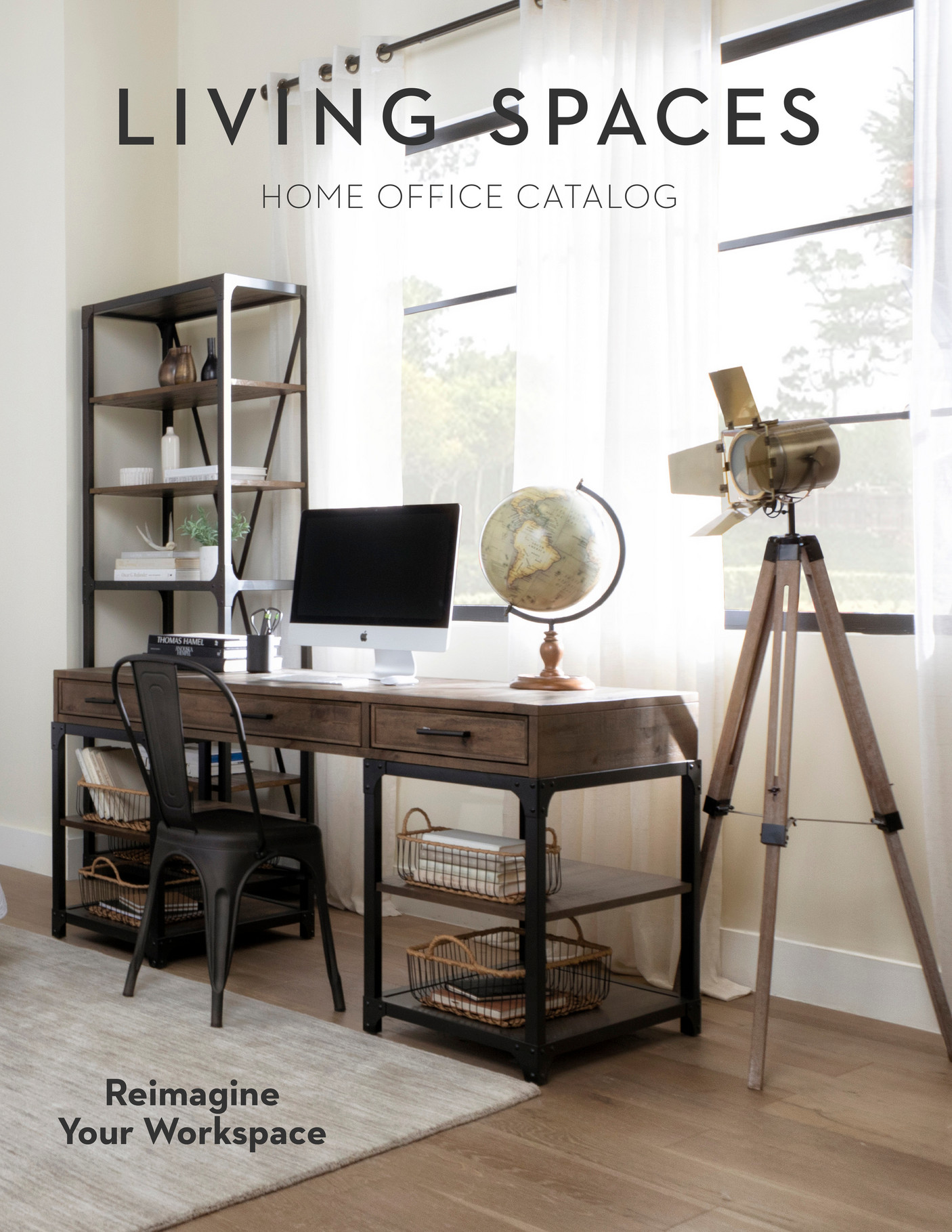The image, featured on the front of the Living Spaces home office catalog, showcases a bright, pristine room designed with a modern, minimalist aesthetic. In the foreground, there is a stylish brown wooden desk with metal accents, positioned directly in front of two large windows adorned with open white curtains that allow a glimpse of the outside vegetation and trees. A sleek metal chair is pushed into the desk, which hosts an Apple Mac computer screen and a brown globe. 

To the left of the desk stands a tall wooden bookshelf with metal accents, decorated with various items, including bottles in white, bronze, and black. On the right side of the room, there is a wooden and metal decorative tripod light, erroneously described as a telescope. The floor is a light brown wood, partially covered by a light gray rug. Text on the image reads "Living Spaces Home Office Catalog" at the top and "Reimagine Your Workspace" in dark gray at the bottom left corner, highlighting the catalog's theme of rethinking and refreshing office spaces. The overall ambiance is professional, clean, and welcoming, indicative of a well-designed workspace in a home setting.